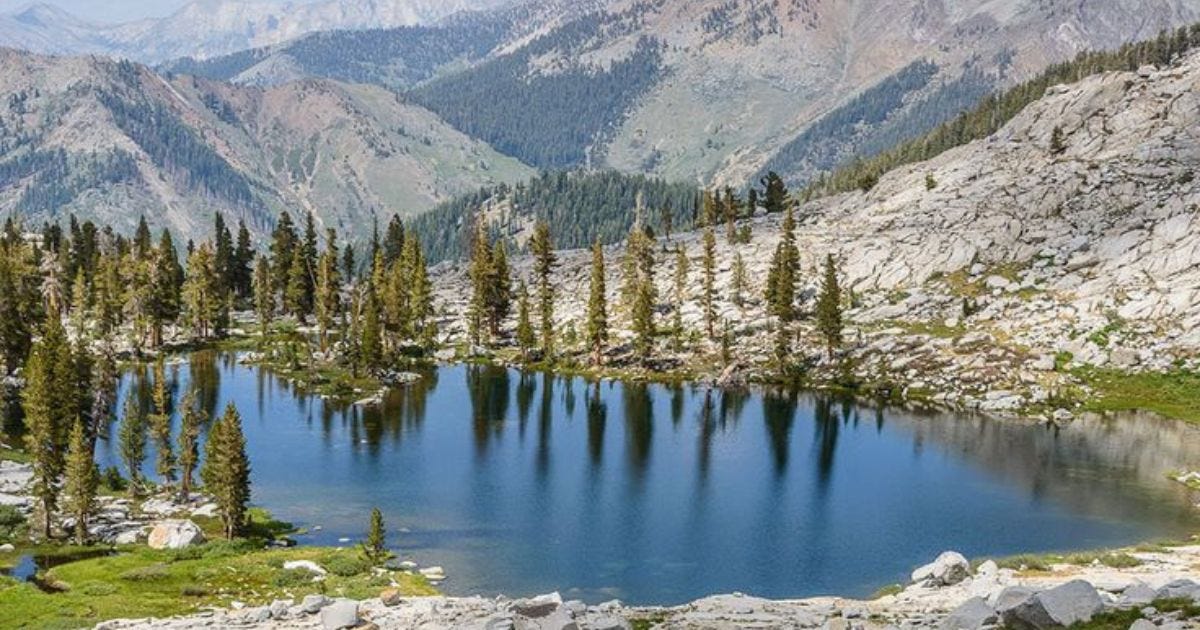The image captures a serene nature scene in a forested mountain area on a sunny day. In the foreground, there is a small, opaque pond reflecting the surrounding tall pine trees, which resemble Christmas trees in their lush, green appearance. The pine trees vary in size, creating a layered effect around the pond, and there is a mix of grass and light gray rocks scattered throughout the scene. To the right of the pond, a snow-dusted hill enhances the wintry atmosphere. In the background, towering mountains stretch up to the top edge of the picture, effectively blocking the view of the sky. The mountains display a mosaic of grassy areas, rocky outcrops, and clusters of trees, completing the tranquil and picturesque wilderness setting.